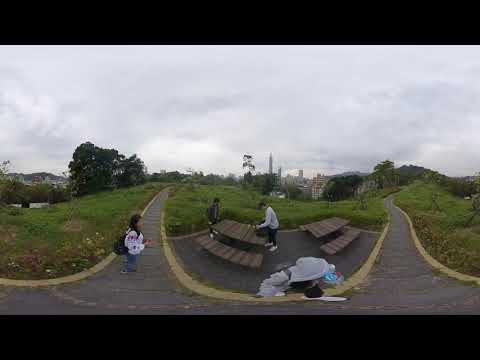This photograph captures a vibrant outdoor garden or hillscape, viewed through a fisheye or 360-degree panoramic lens, giving the image a distinct curved and bulging perspective. At the center, there are two narrow, grey paved paths bordered in light yellow that converge at the end of the image. On the left path, a woman is seen walking, identified by her black backpack, white long-sleeved jacket, and blue pants.

In the middle of this beautifully green scene, where lush grass and various plants flourish, stand two wooden picnic tables. By one table, two individuals are positioned; one wears a white shirt, black pants, and white shoes, while the other is dressed in a gray shirt. There is also a pile of indistinct light-colored objects next to the picnic setup. The scene extends to the distant background, showcasing some trees, rolling hills, and mountains. Above, the sky is a mix of scattered clouds and patches of blue, creating an overcast ambiance. The image is infused with the sense of space and natural beauty, emphasizing the rich greenery and the serene, outdoor setting.